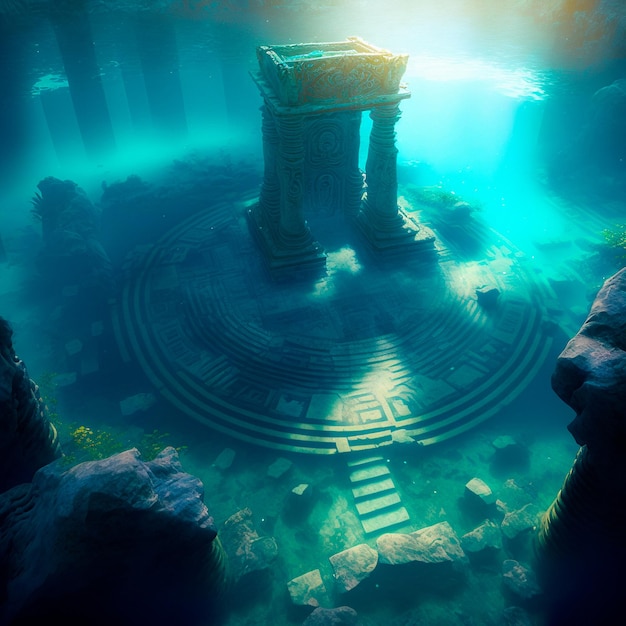The image is a highly detailed, AI-generated or digitally created depiction of an underwater ruin, likely inspired by the mythical lost city of Atlantis. In the center, there is a circular altar made of concrete or stone, featuring intricate geometric and square carvings along its sides. Steps lead up to this altar, which supports a small structure with four stone pillars topped by a rectangular, crown-like feature. Surrounding the central structure, scattered across the sea floor, are numerous gray boulders and stones. Additional tall, dark silhouettes of pillars can be seen in the background. Light penetrates the aqua-blue water from the upper right corner, casting an ethereal glow on the scene, which contributes to its fantasy world aesthetic. A few grass plants and bubbles complete the realistic underwater ambiance of this artistic representation.